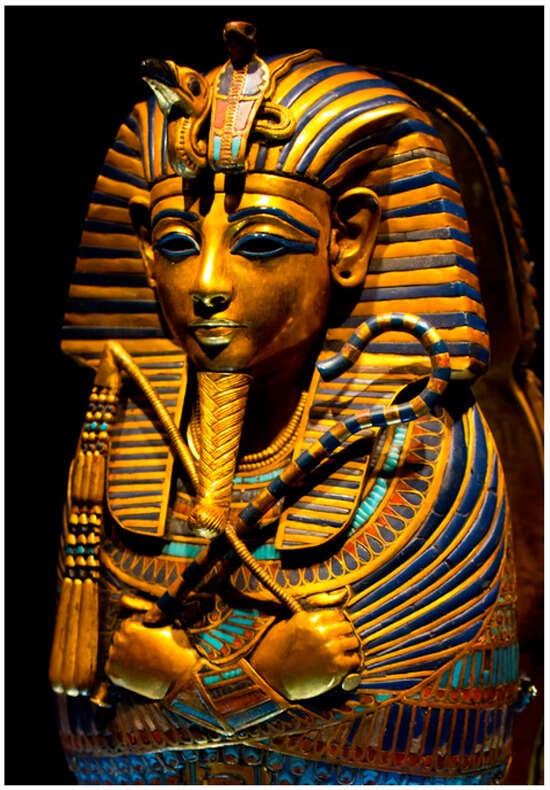This image captures the exquisite sarcophagus of King Tutankhamun, the renowned ancient Egyptian pharaoh. The sarcophagus features intricate blue and gold horizontal stripes that adorn both his elaborate headdress and his regal attire. Prominently, the headdress showcases a vulture and a cobra, symbolizing protection and sovereignty. The pharaoh's serene face is accentuated with blue makeup and meticulously painted blue eyebrows. His arms are crossed over his chest, holding two symbolic objects: a straight rod with horizontal striations and a hooked rod reminiscent of a shepherd's crook, both echoing the blue and gold theme. The striking image reveals a long, intricately braided beard extending from his chin. Furthermore, the sarcophagus boasts additional red and light blue details lower down, enhancing its visual grandeur. A dark backdrop serves to highlight the vivid colors, making the ancient craftsmanship even more compelling.